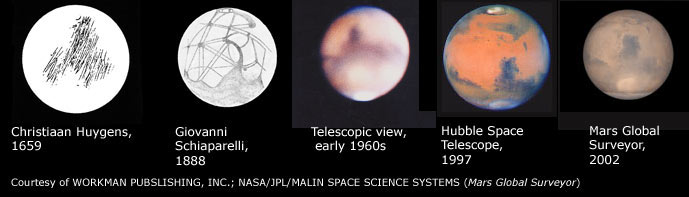This horizontal rectangular image has a black background and showcases five different views of Mars, ranging from 1659 to 2002. Each of the five circles represents a different era of Mars observation. From left to right:

1. The first circle, labeled "Christian Huygens, 1659," features a white circle with black scribbles.
2. The second circle, labeled "Giovanni Schiaparelli, 1888," shows a white circle with black lines depicting the first drawn canals on Mars, reflecting Schiaparelli's observations.
3. The third circle, "Telescopic View, early 1960s," displays a blurred image of Mars, highlighting the telescopic capabilities of that time.
4. The fourth circle, "Hubble Space Telescope, 1997," presents a clearer, colorful image of Mars, with blue and orange hues, demonstrating the advanced imaging power of the Hubble Telescope.
5. The fifth and final circle, "Mars Global Surveyor, 2002," shows a clear, detailed view of Mars with blue and beige tones.

At the bottom of the image, it states, "Courtesy of Workman Publishing, Inc., NASA, JPL, Malin Space Science Systems, Mars Global Surveyor," indicating the sources and contributions to these Mars images. The diagram effectively illustrates the progression of our observational capabilities and understanding of Mars over several centuries.